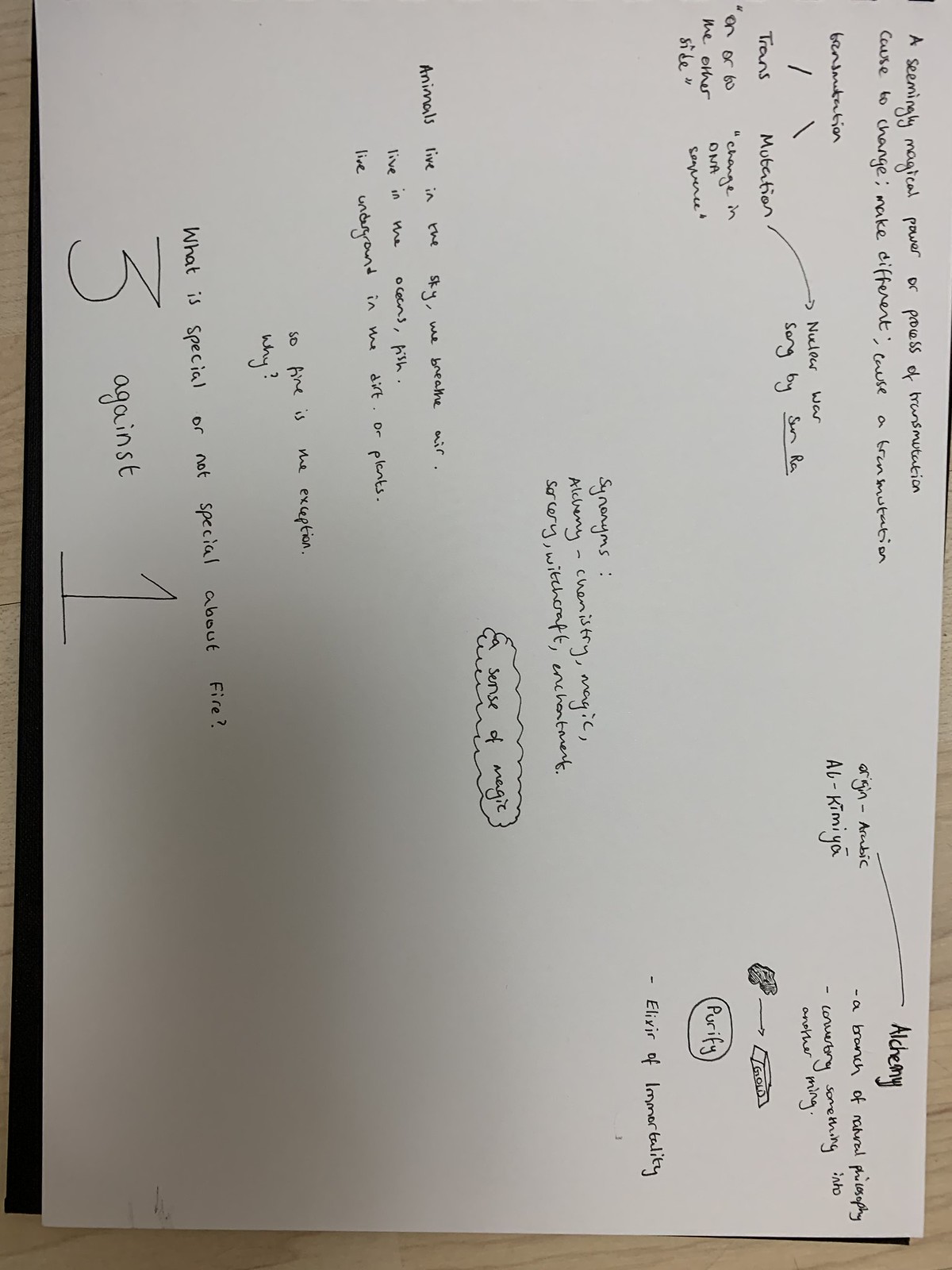A rectangular photograph depicts a white sheet of paper placed sideways on a flat brown wooden surface. The sheet, positioned so that its top points to the right and its bottom to the left, is filled with handwritten notes made in pen or pencil. The notes cover a variety of subjects related to the concept of transmutation and alchemy. Detailed inscriptions include phrases such as "a seemingly magical power or process of transmutation," "caused to change, make different, cause a transmutation," and descriptions of "mutation, change in DNA sequence." The notes also reference "Nuclear war, song by Sun Ra," and note the "Origin, Arabic, alchemy" with a definition, "alchemy, a branch of natural philosophy." Additionally, a simple drawing illustrates a rock with an arrow pointing towards a gold bar, symbolizing the process of alchemical transformation. The meticulous and diverse annotations suggest a deep exploration of both scientific and mystical aspects of transmutation.